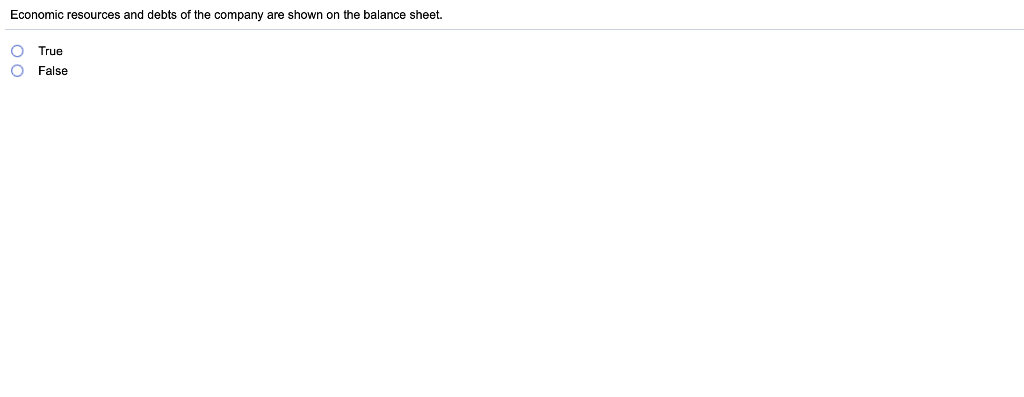This image is a minimalistic screen capture featuring an informative message within a predominantly white background. At the center of the image, black text reads, "Economic resources and debts of the company are shown on the balance sheet." Below this text, a very pale, horizontal light gray line spans the entire width of the screen, offering a subtle separation. Positioned beneath this line are two faint gray circles aligned vertically on the left side of the screen. Adjacent to the first circle on its right is the word "True," while the second circle below it has the word "False" to its left. Both words are rendered in black text with only the initial letters capitalized, providing a clean and straightforward look.